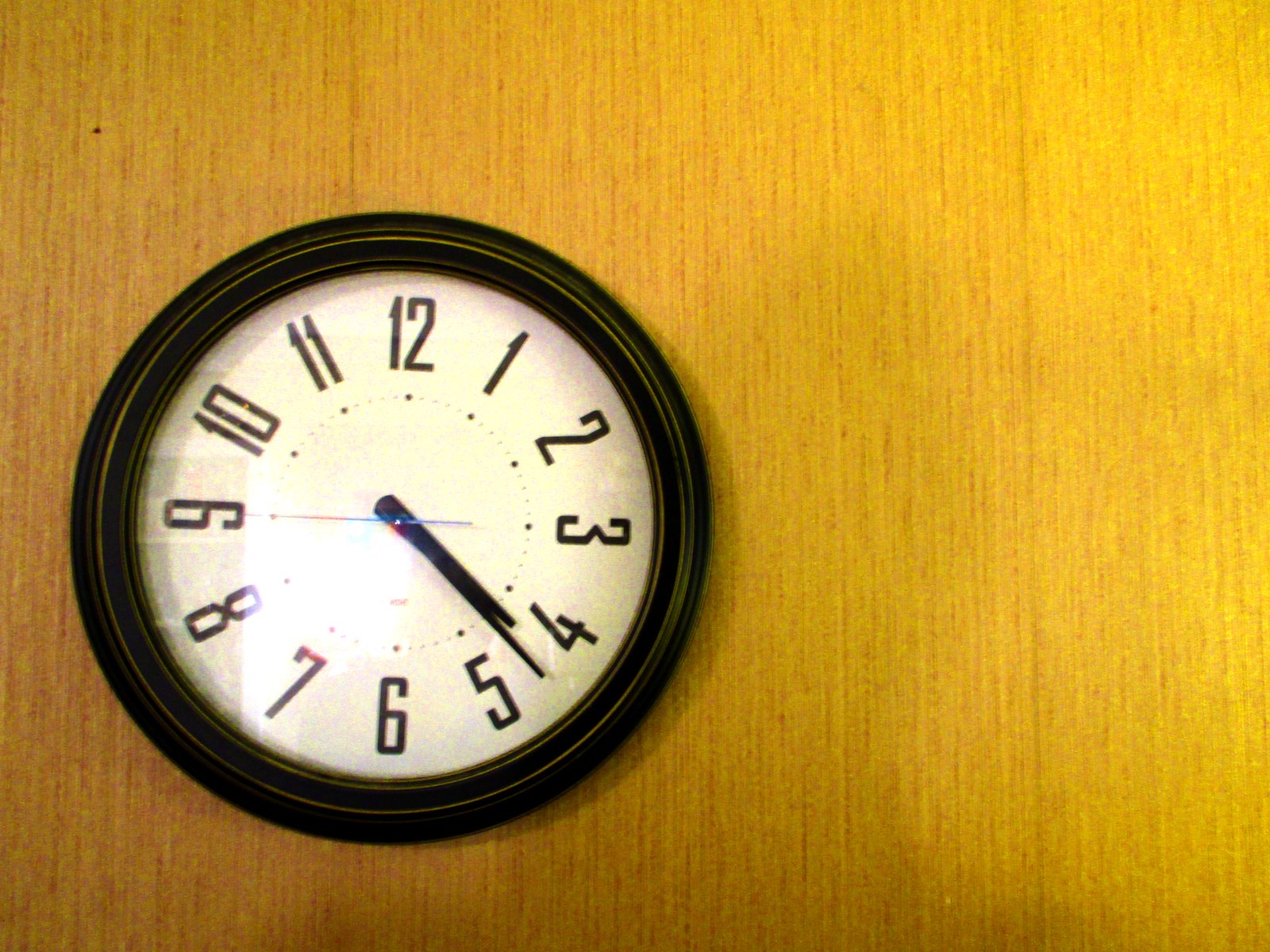This image captures a detailed view of an analog wall clock mounted on a light beige wooden wall featuring very faint brown streaks. The clock is circular with a prominent black frame accented with a very thin gold or yellow edge on the inner side. Its white dial is contrasted by large black numbers and hands, while the thin second hand is distinctly blue. The glass cover over the dial reflects light, adding a subtle gleam to the scene. The clock is positioned on the left side of the image and displays the time as 4:22. Small dots circumscribe the dial, marking the minutes, with slightly larger circles for the hour positions. The camera angle suggests a slightly downward view, almost as if the viewer is looking at the clock from a standing position over it.